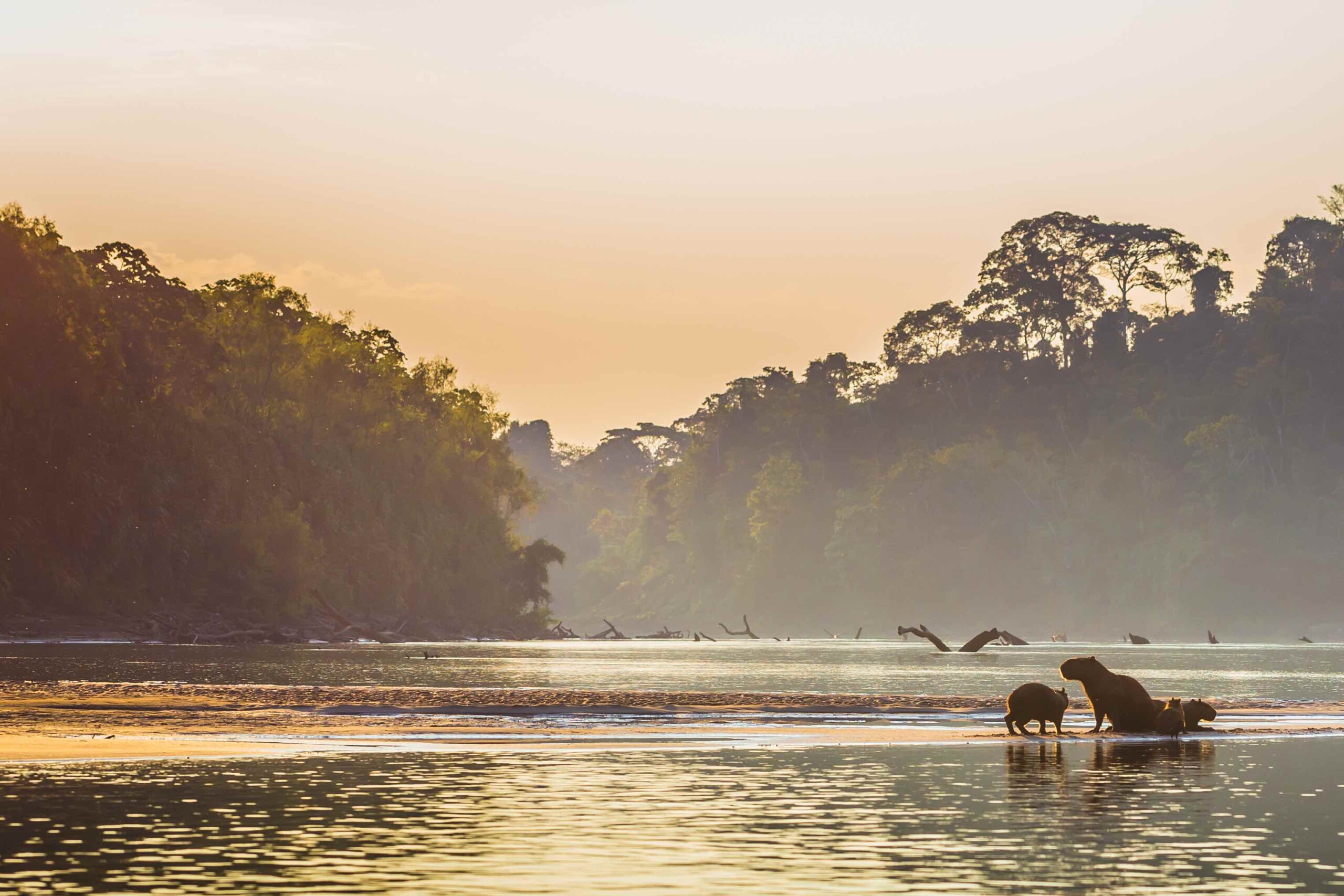The image captures a serene river landscape framed by dense greenery, with towering dark green trees lining both the left and right sides of the wide, rectangular frame. The sky, painted in soft hues of orange and gray, suggests either sunrise or sunset. The calm, dark-gray water, reflecting the sky's colors, stretches from the bottom of the image towards the center, creating a tranquil scene with a few tree limbs protruding from its surface in the distance. Near the bottom right corner, a family of animals, presumably beavers, huddles close to a sandbar. The adult beaver, accompanied by smaller ones, blends into the shaded environment, their short-haired, rounded forms silhouetted against the backdrop. The water, gently rippling, reflects the quiet beauty of the wilderness, hinting at a forested expanse beyond, filled with verdant trees.